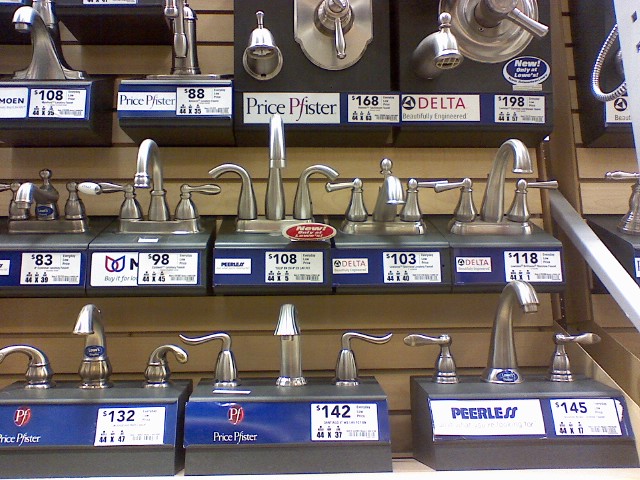This photograph, taken in an indoor home improvement store, showcases a display of various faucets and shower heads mounted on a light brown, horizontally-palleted wooden wall. The display is organized into three distinct rows. The bottom and middle rows feature primarily bathroom faucets, each with two handles and a curved spout, all in a stainless steel or pale gray color. Each faucet sits on an individual gray display stand, accompanied by a blue banner that bears the brand name and price tag on a white rectangular patch. Brands visible include Peerless, Delta, and Price Pfister, with prices ranging from $83 to $145.

On the top row, to the left are two faucets, while the right side presents two black boxes with faucets and knobs that can twist in a complete circle. The middle row, centrally located in the photograph, exhibits five faucets in similar styles, each with left and right handles and a central spout. The bottom row features three faucets, maintaining the same design but in varying sizes. Above these rows, shower heads and spouts for showers are displayed on similar gray stands. The entire scene is framed within a square photograph, capturing the well-organized and detailed presentation of bathroom fixtures.